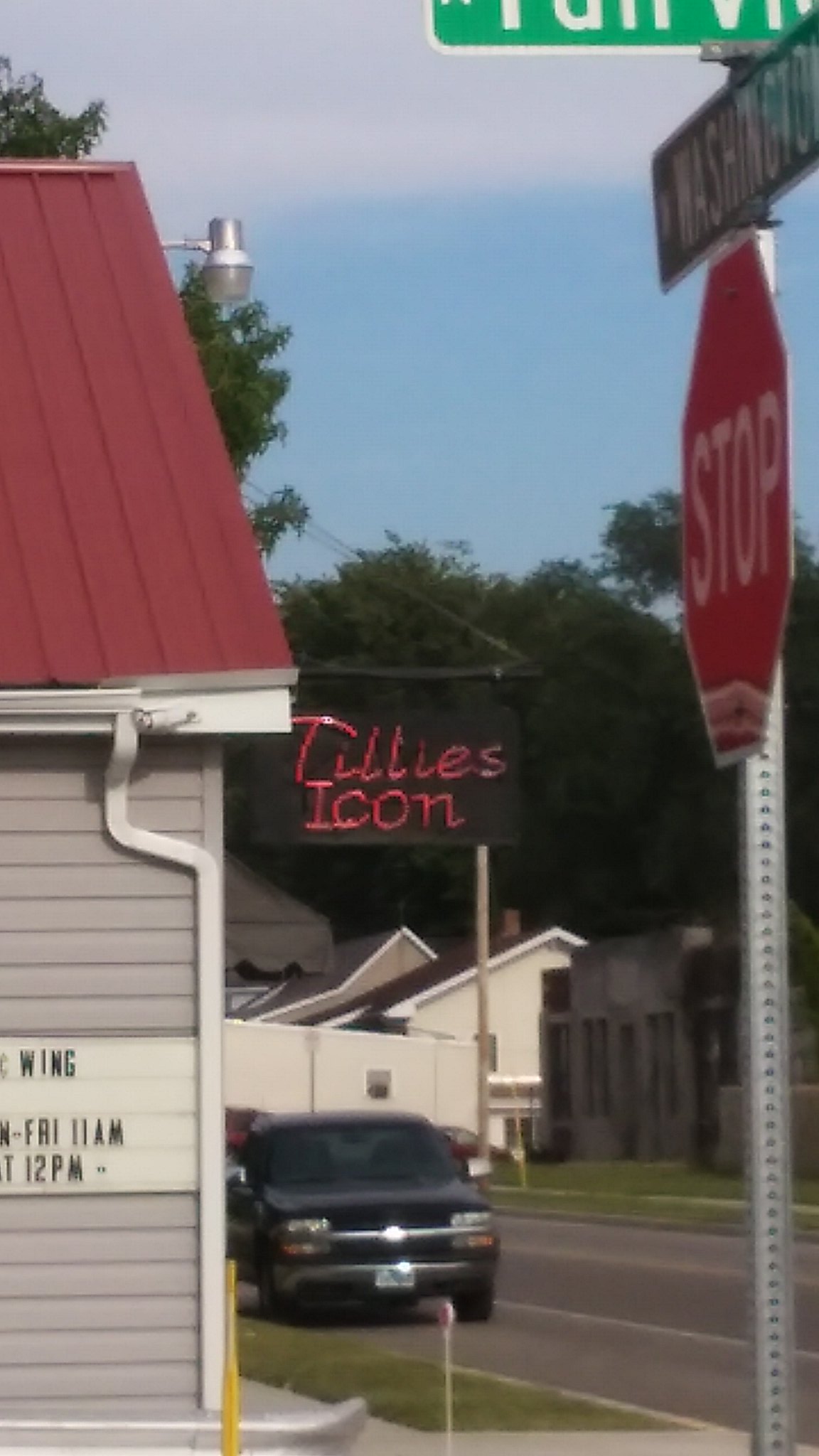This photograph captures a slightly blurred street view taken at an intersection. Prominently in the foreground, there is a red stop sign with white font, mounted on a perforated metal pole. Affixed to the top of the stop sign are two street signs, both green with white font; one reads 'Washington,' while the top of the other sign is cut off and unreadable. A grey wooden building with white gutter drains and a red slatted roof, possibly metal, is situated on the left. This building features a marquee sign with black letters spelling out 'Tilly's Icon' on a black background, and a white sign board with partially legible text, mentioning 'wing, Monday through Friday at 11 AM.' 

In the intersection, a black vehicle, likely an SUV, is driving towards us. The scene also shows a partial glimpse of sidewalk, some of the road, and patches of green grass. Further in the background, there are a couple of houses extending down the road, along with tall green trees. The sky overhead is blue with clear white clouds. On the left side, there is a visible street light, adding to the suburban atmosphere of the image.